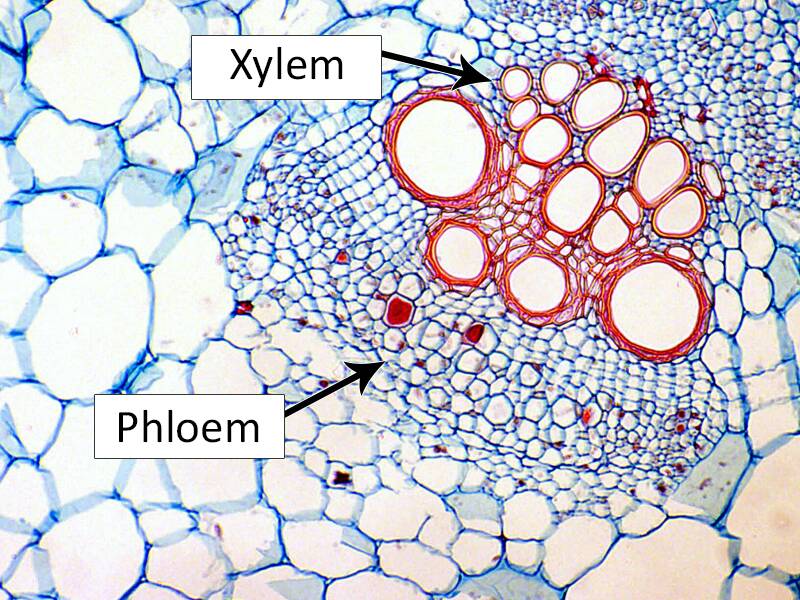This detailed image appears to be a highly magnified biological diagram, possibly from a textbook. The central focus of the image includes various colored shapes and annotated sections. Prominently, two types of structures are highlighted: a cluster of red circles with white interiors and a periphery comprising blue circles, also with white interiors. The red circles in the middle are labeled with a white box and black text that reads "Xylem," with an arrow pointing directly at them. Similarly, a different white box with black text labels the blue circles as "Phloem," with another arrow indicating these structures. The diagram spans the entire page and features a meticulous arrangement of these colored circles, suggesting an educational purpose to illustrate the distribution of xylem and phloem in plant tissue or cellular structures.